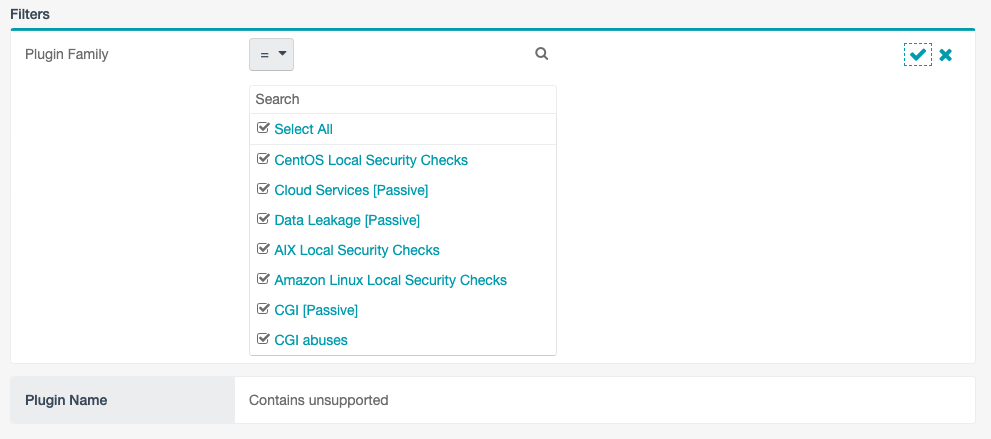**Detailed Descriptive Caption:**

The image is a horizontally rectangular screenshot featuring a primarily white background with a light gray border. At the top left corner of the screenshot, the text "Filters" is displayed in bold black. A thin teal green horizontal line separates the gray border from the central white background. Below this line, on the left side, the label "Plug-in Family" is visible.

An adjacent search field is provided, under which there is a vertical list of items with all boxes checked. This list includes options like "Select All," "CentOS Local Security Checks," "Cloud Services Passive," "Data Leakage Passive," "AIX Local Security Checks," "Amazon Linux Local Security Checks," "CGI Passive," and "CGI Abuses."

Beneath these options, still on the left side, the label "Plug-in Name" is displayed. Directly across from this label is a white field containing the text "contains unsupported". The design elements appear neatly aligned, providing a clean and organized user interface.